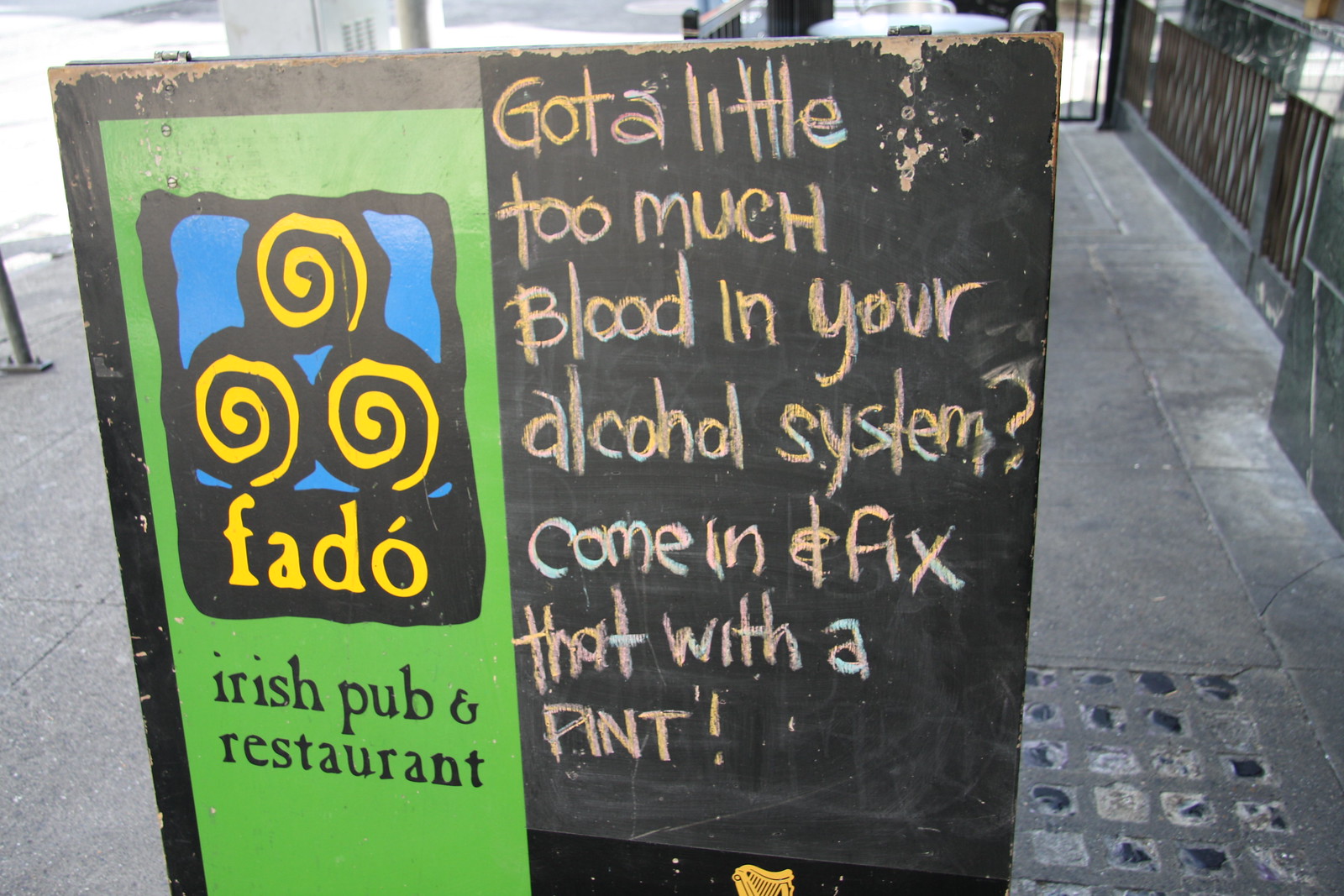This rectangular photograph depicts a city street scene featuring a prominent sign standing on the sidewalk, which is partially covered with snow, indicating it may have been taken during the wintertime. The daytime lighting suggests it was captured during daylight hours. The sidewalk itself is a mix of cobblestones and regular concrete, with an iron and marble railing visible on the right side. The sign, likely advertising a nearby establishment, is divided into two distinct sections. The left side features a green background with yellow swirls on a blue backdrop and includes the text “FADO” with an accent, alongside “Irish Pub and Restaurant” written in yellow. The right side resembles a chalkboard and carries a playful message written in orange, blue, and pink chalk: "Got a little too much blood in your alcohol system? Come in and fix that with a pint." The humorous text, combined with the pub logo and details, suggests it is an inviting call for patrons to visit the Irish pub and restaurant likely situated nearby.